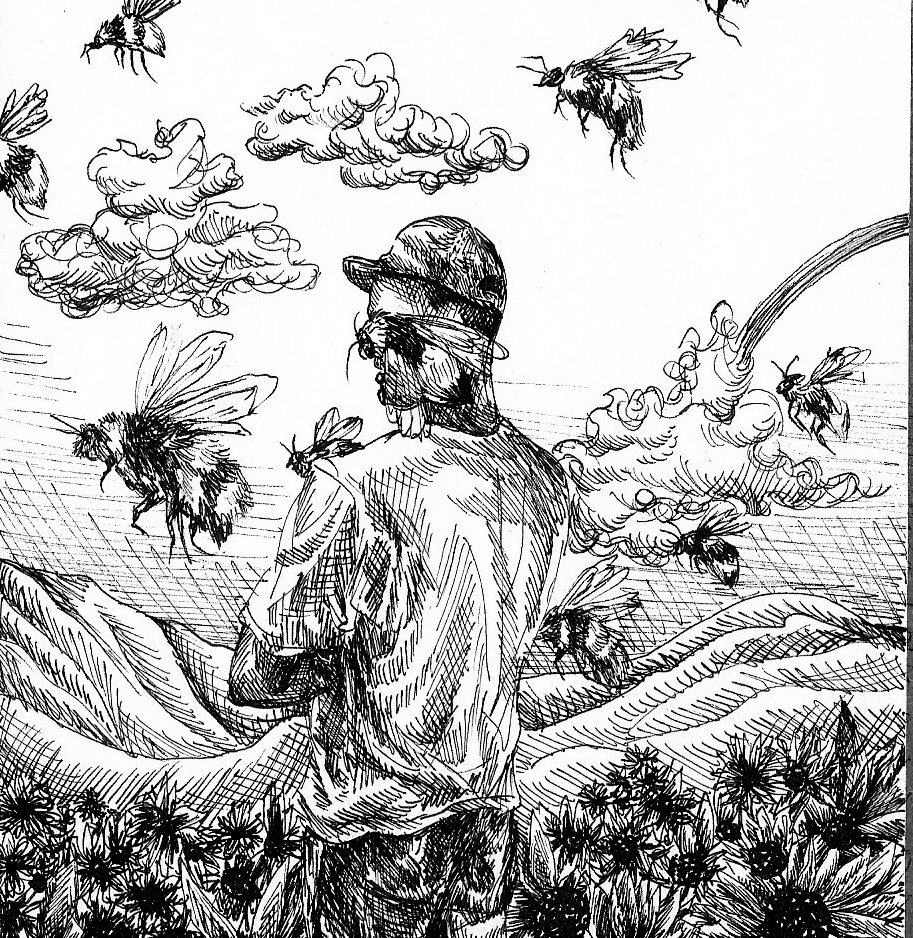A detailed black-and-white pen-and-ink drawing depicts a man sitting in a large, flower-dotted field, surrounded by giant, fluffy bees. The man, shown from the waist up, is wearing a sideways-facing baseball cap and a t-shirt. He appears relaxed, with his legs slightly outstretched amidst the hills and fields that form the background. The bees are extraordinarily large—almost the size of his head—and are characterized by their hairy bodies, six legs, and antennae. The scene is framed by scribbly, cloud-like formations in the sky, adding to the whimsical yet intricate nature of the piece.